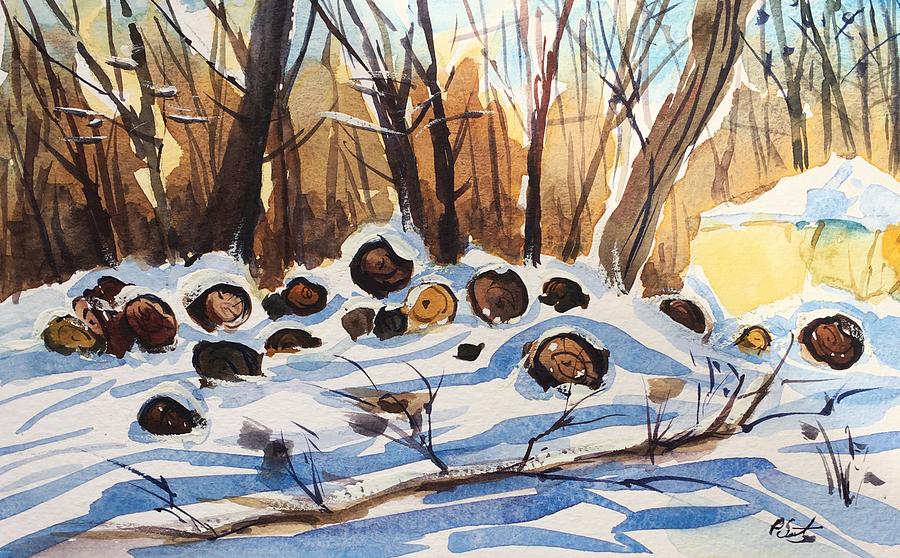This watercolor painting, done in an impressionistic style with curvy lines and shapes, depicts a serene winter forest landscape. Prominently in the foreground lies a fallen brown tree, its branches sprawled across the snow-covered ground. Behind this, several dark brown logs are neatly stacked and partially buried in the heavy white snow, suggesting they have been cut and arranged methodically. The snowy scene is interspersed with streaks of blue paint, adding depth to the wintry tableau. In the background stand numerous leafless, colorless trees, subtle yet distinct with their wiry branches reaching skyward. Rays of sunlight filter through these trees, enhancing the natural beauty of the scene.

On the right side of the composition, a yellow-tinged structure, possibly a tent, peeks through the snowy expanse, its roof also capped with snow. This structure adds a splash of color to the predominantly monochromatic palette. The artist's indistinct signature, beginning with a "P" and seemingly ending in "S," can be found in the bottom right corner of the painting. Overall, this simple yet detailed watercolor captures a quiet, snowy woodland moment with a delicate and meticulous touch.